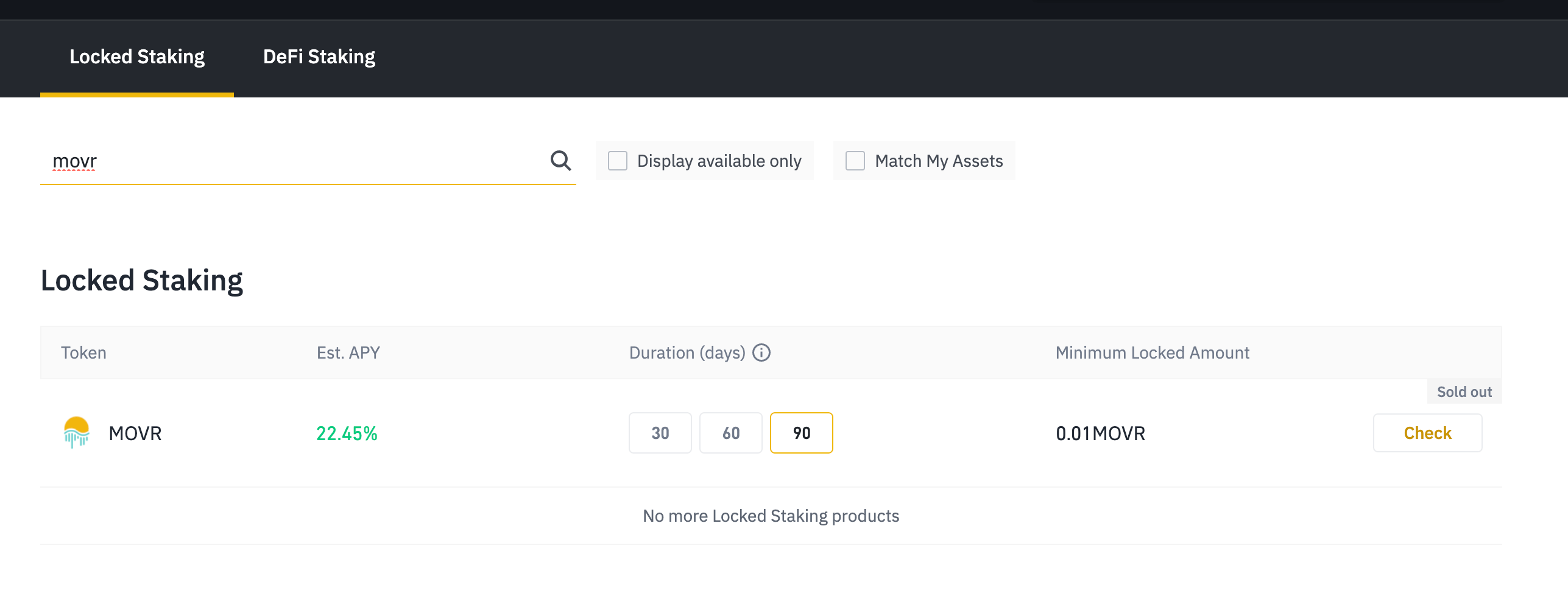Screenshot of a website featuring a user interface with financial options. At the top, a black banner spans the width of the screen, though the website's name is not visible. The main area displays two navigation options: "Locked Staking" and "DeFi Staking." Occupying the most prominent space on the page, the heading "Locked Staking" is shown in large, bold font. Below this, the specific token "MOVR" is highlighted, and the Annual Percentage Yield (APY) for this token is prominently displayed in green text at 22.45%. The interface provides a choice for the duration of the staking period, offering options of either 360 days or 90 days, with the 90-day option currently selected. At the bottom of the screen, a message states, "No More Locked Staking Products." The underlying background is minimalistic, rendered entirely in white except for the black top bar, offering no additional layout or design features of the website itself.